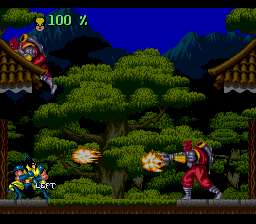An image captures the screen of an old-school video game, likely from the early era of video games or arcade machines. The background showcases a lush scene with a tree adorned with vibrant green leaves and surrounding shrubbery. In the distance, a picturesque landscape of mountains under a clear blue sky adds depth to the setting. On both the left and right sides, Japanese pagodas with distinctive tiled roofs frame the scene, adding an Eastern aesthetic.

On the left side of the image, a ninja warrior clad in red and grey is seen scaling the roof of a pagoda, embodying stealth and agility. Below, another character stands poised in a fighting stance, donning a striking blue and yellow outfit. This character's readiness suggests an impending battle.

To the right, near the bottom of the image, another ninja-like figure, dressed in red with grey boots or leggings, is captured in the act of firing a weapon, adding an element of action and excitement to the scene. This character's aggressive posture contrasts with the tense readiness of the blue and yellow warrior.

In the top-left corner, digital green numbers display "100%," possibly indicating player health or game status, completing the image with a nostalgic touch reminiscent of vintage gaming interfaces.